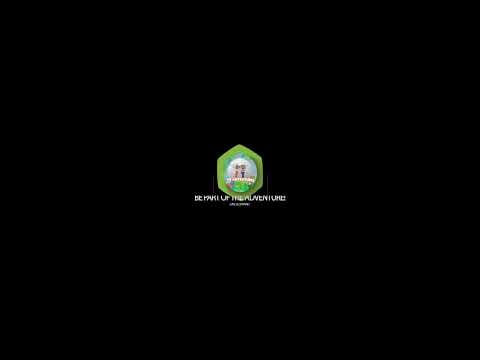The image depicts a company logo set against a solid black background. The logo resembles a small emblem or badge, primarily pentagonal but sometimes perceived as diamond-shaped. The outer border of the logo is green, reminiscent of grass. Inside the logo, there is a scene featuring two human figures facing each other, standing against a blue background that evokes a sky-like feel. These figures are positioned above a yellow banner. Beneath this scene, there are two lines of text in a foreign language. The upper line is slightly larger but still not legible, while the smaller text beneath it reads, "be part of adventure," though the exact wording is difficult to decipher.